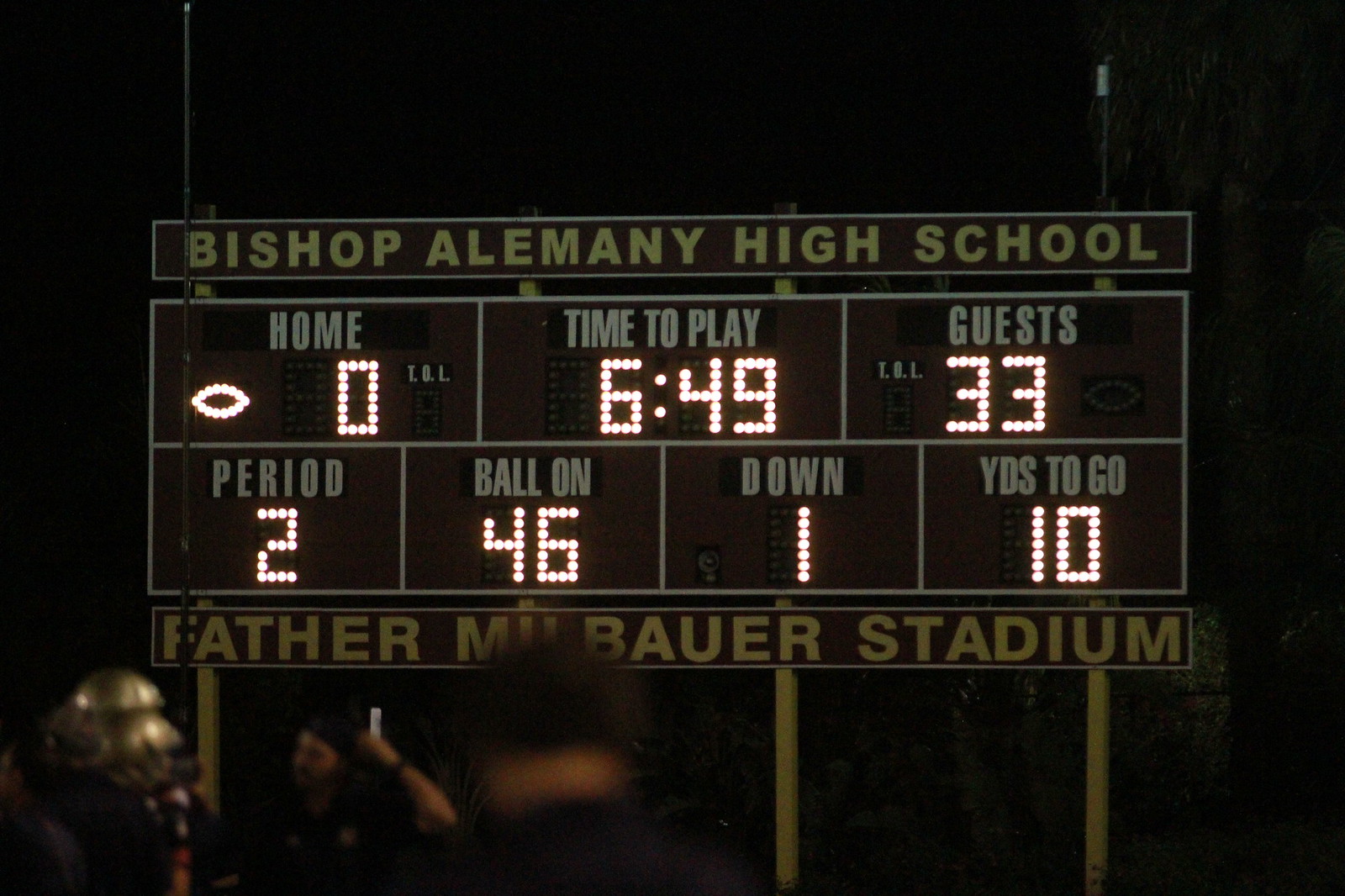This is a nighttime photograph of a high school football game scoreboard at Father Milbauer Stadium, home to Bishop Alemany High School. The scoreboard, supported by three yellow poles, features bold yellow lettering at the top that reads "Bishop Alemany High School" and "Father Milbauer Stadium." The black scoreboard is illuminated by round light bulbs, creating a bright display of game metrics. The home team is currently scoreless, with a score of 0, while the guests are leading with 33 points. The time remaining in the second period is 6:49. Additional game details are displayed, indicating that it is the first down with the ball positioned on the 46-yard line and 10 yards to go. The vivid white lights on the scoreboard contrast against the dark night sky, and in the blurred foreground, a few gold-helmeted football players and coaches can be faintly seen.